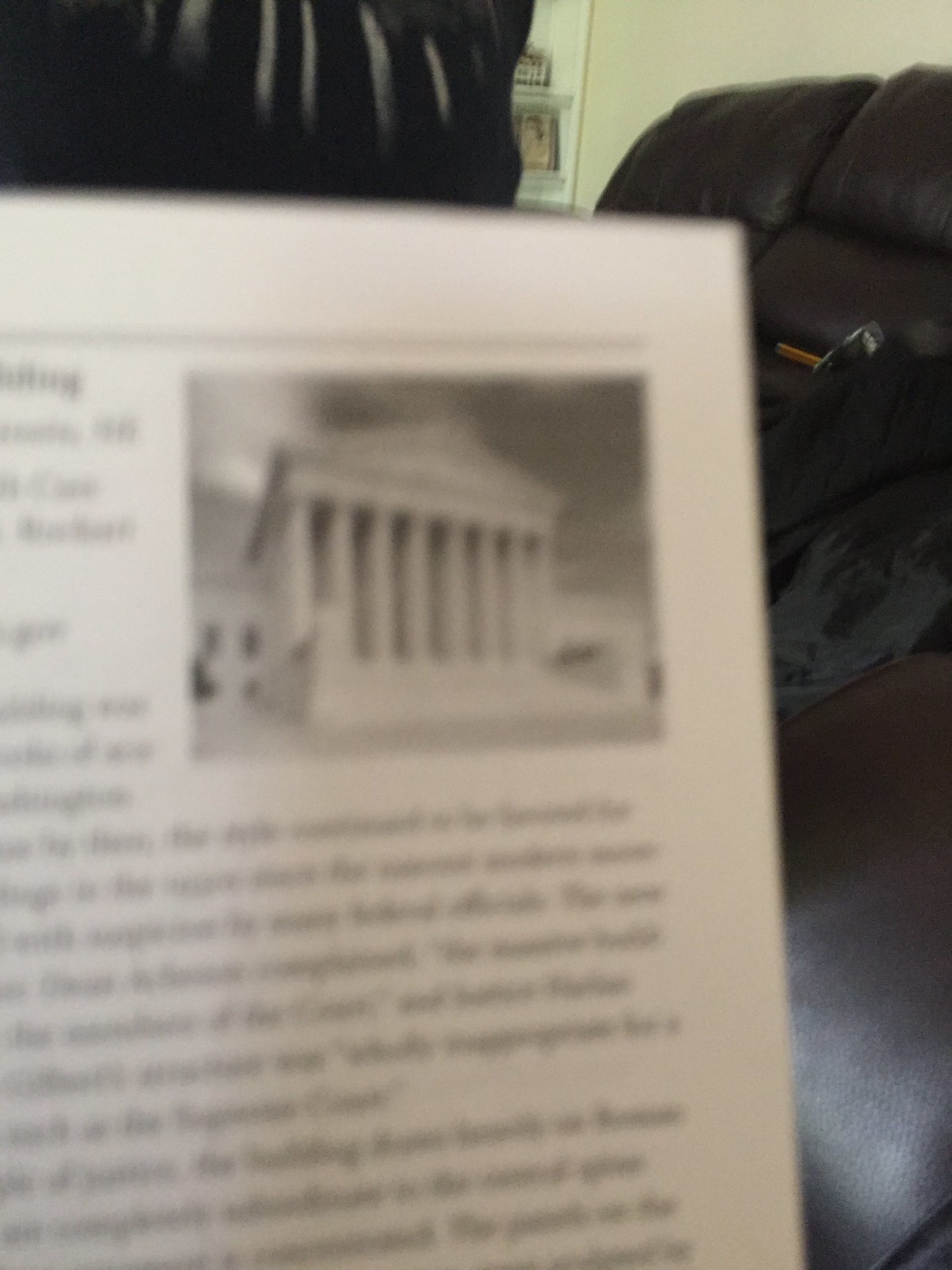A very blurry color photograph features an open book prominently in the left foreground. The book's pages contain writing that is indiscernible due to the blur. Attached to the top right corner of the book is a black and white photograph depicting a Roman-style building characterized by several pillars at the front and a staircase leading up to it. The background is somewhat cluttered with unidentifiable black objects, lending an air of mystery to the scene. On the right side of the image, there appears to be a large, overstuffed leather couch. Further adding to the complexity, the top left of the image contains another black object that remains a mystery. The entire setup is against a backdrop of a white wall, which displays a hanging picture that is indistinct and unclear to the viewer.